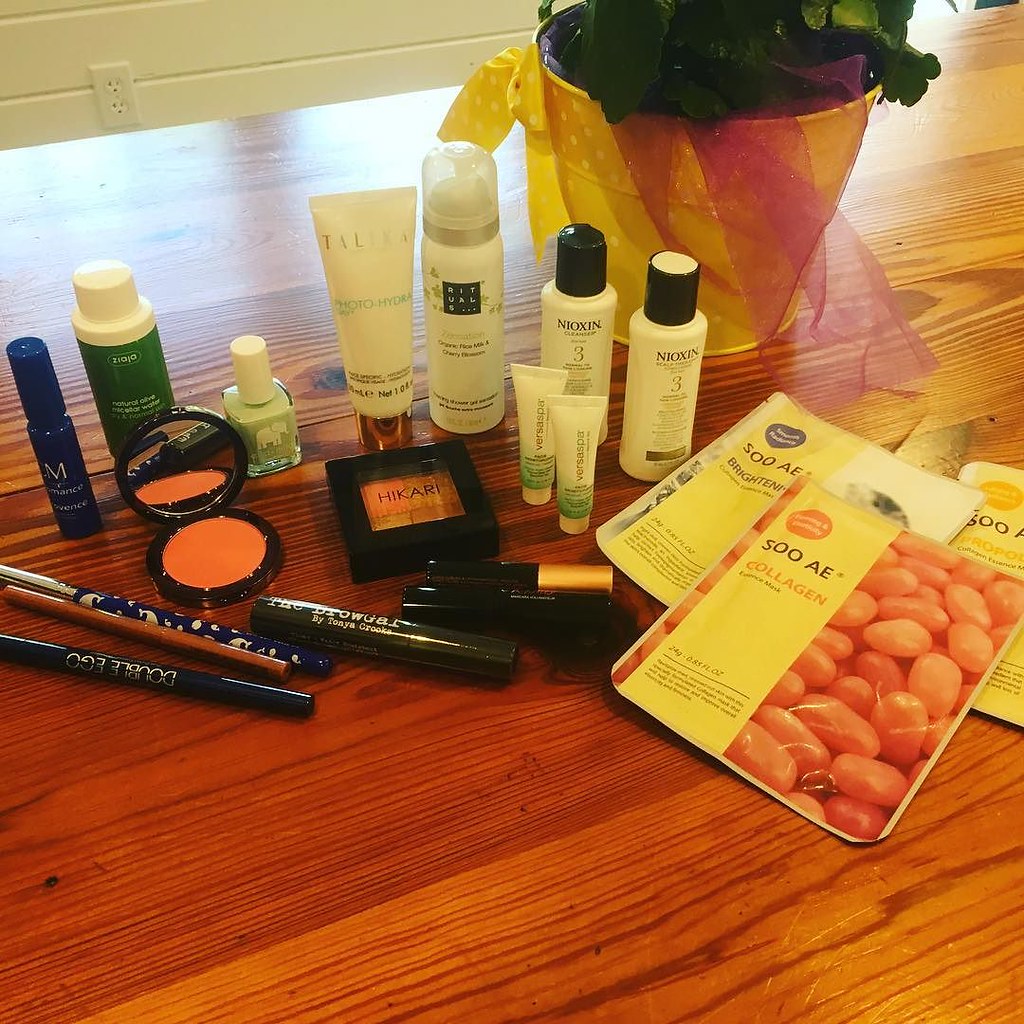A collection of beauty products is spread across a reddish-brown wood tabletop, showcasing a rich wood grain pattern. Among the items, a yellow bucket with green leafy plants is adorned with a purple ribbon or lace at the top. To the right, three SoAE face masks, framed with a yellow border on the left side, prominently display labels such as "collagen" and "brightening", while the text on the third mask is partially obscured.

To the left of the face masks, various bottles are arranged. Notably, two white bottles with black lids are branded with "Nioxin". Nearby, shorter tubes with white and green designs are labeled "Versapar". A taller canister with a spray top and a clear lid features the name "Ritual 5".

Further in the arrangement, a white tube with a bronze-colored cap displays "Photohydra Talyxa". Among the makeup containers, there is a black square item branded "Hikari" and a black circular compact with a mirror containing orange powder. A green nail polish with a white cap marked with an elephant emblem shares space with another green bottle with a white cap labeled "Zeotia". Nearby, a blue bottle with a blue cap reads "M Performance".

Several eyelash pencils in blue, brown, and black hues are interspersed among the items, accompanied by black mascara cases labeled "the Brow Gal by Toni Crook." Additionally, two other black mascara tubes are present, one of which features a bronze-colored cap.